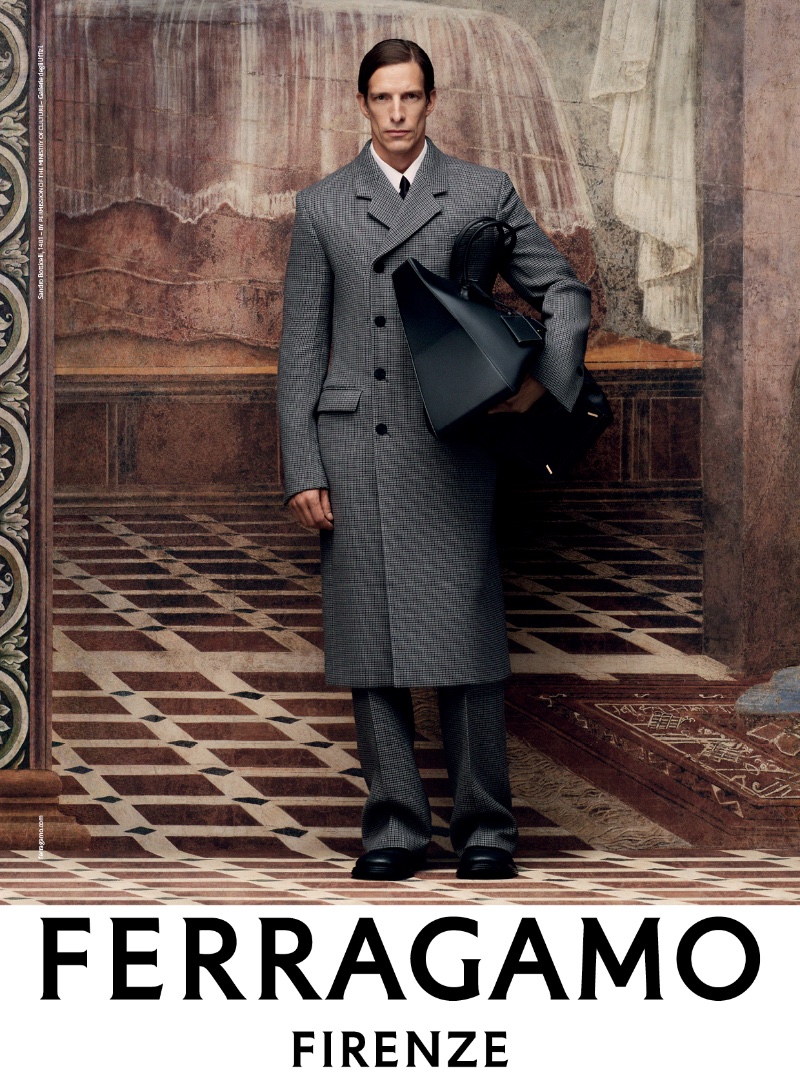This professionally staged full-color photograph, featuring a young Caucasian man, serves as an advertisement for Ferragamo. The image itself is square and lacks a border. Dominating the bottom of the picture in bold black capital letters, "FERRAGAMO" is prominently displayed, with the word "FIRENZE" in smaller font beneath it. 

The man is impeccably dressed, wearing black shoes, gray slacks, a white shirt and black tie, complemented by a long, knee-length gray overcoat. His hair is neatly combed to the side, and he carries a large black leather satchel, held securely under his left arm by its handles.

The setting appears to be an elegantly decorated indoor space with mid to dark brown walls and a marble tile floor in shades of white and brown. A decorative column stands to his left, contributing to the sophisticated ambiance, which might evoke the feel of a museum or a high-end gallery.